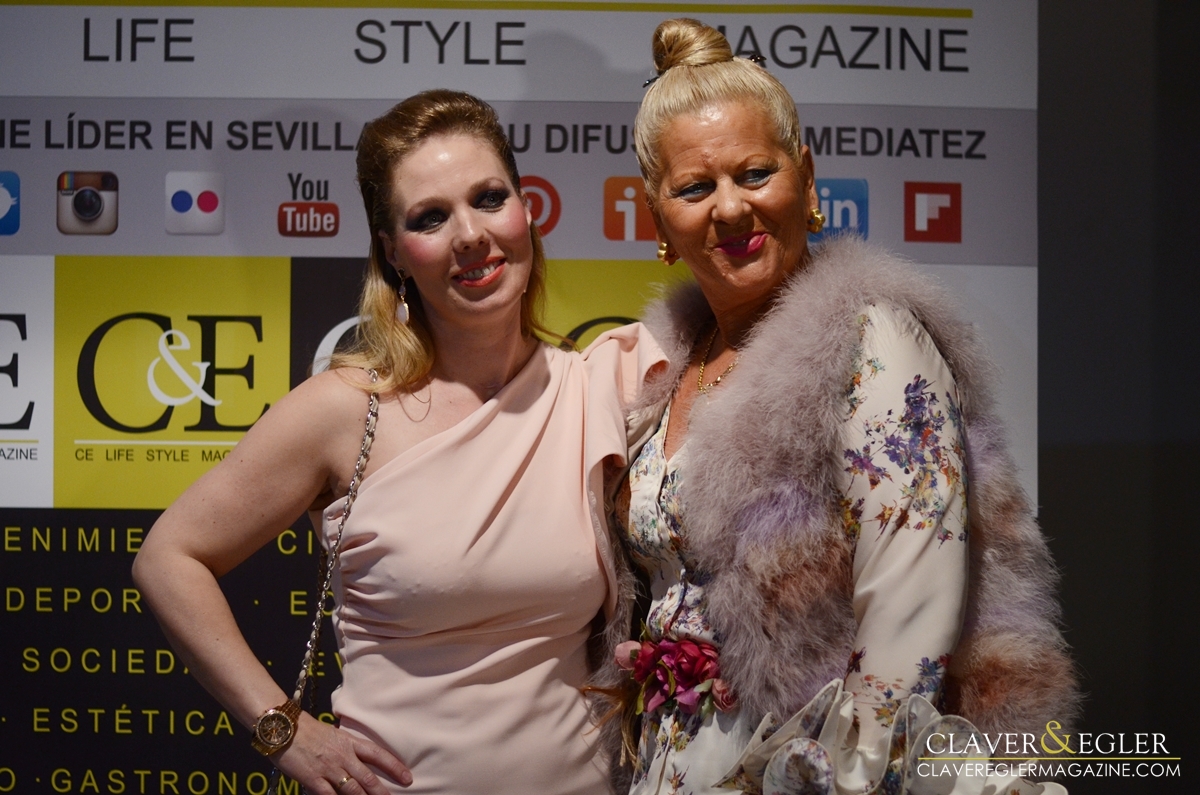The photograph features two women, elegantly dressed, standing in front of a white backdrop bearing the text "Lifestyle Magazine" and various social media logos for Instagram, Twitter, YouTube, and Pinterest. Below this text are yellow squares with the black letters "C" and "E," followed by "CE Lifestyle Magazine." 

The woman on the left appears younger and is wearing an asymmetrical, sleeveless peach dress that wraps around one shoulder. She has a chained strap purse over her shoulder and sports heavy makeup, a watch, and her blonde hair is pulled back. Her arm is comfortably around the woman on the right, who has her hair in a bun and dons a floral top with a fur vest. This second woman, with an older appearance and a deep tan, also has blonde hair and maintains a warm, smiling demeanor.

In the lower right corner of the image, there is a watermark that reads "Claver and Eagler, clavermagazine.com," adding an artistic touch with a watercolor effect. Both women are posing closely together, smiling warmly for the camera.